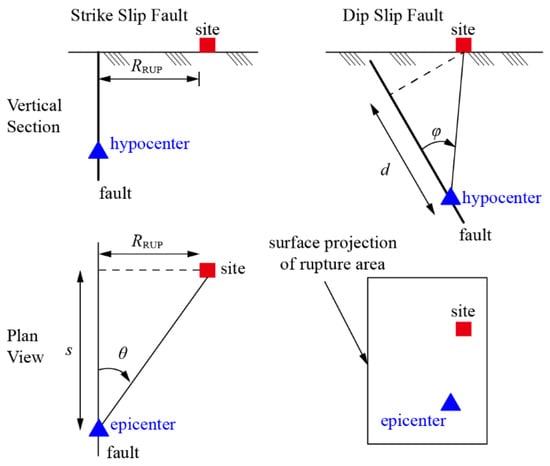The diagram is drawn on a white background and divided into four distinct sections, each illustrating different types of faults and views. The upper sections are labeled "Strike Slip Fault" and "Dip Slip Fault," with the titles in a serif Times New Roman font, though not in all caps. Both sections feature a black fault line with a blue arrow indicating the fault line's direction. 

In each upper diagram, there is a blue triangle representing the hypocenter and a red square representing the site. The left side of the diagram has a vertical section label, clarifying the structure. Adjacent to these sections is a right-angle marker indicating the site, with the epicenter situated next to the blue fault line arrow.

The lower sections are labeled "Plan View" and include a detailed projection of the rupture area. On the right side, the surface projection shows a rectangle outlining the rupture area with a red square denoting the site and a blue triangle for the epicenter. To the left, the plan view depicts a similar setup, where the blue epicenter forms a triangle with the red site marker and the fault line. All text, including "Hypocenter" and "Surface Projection of Rupture Area," is consistently written in Times New Roman font, with important terms such as "epicenter" and "site" clearly labeled in blue and red, respectively.